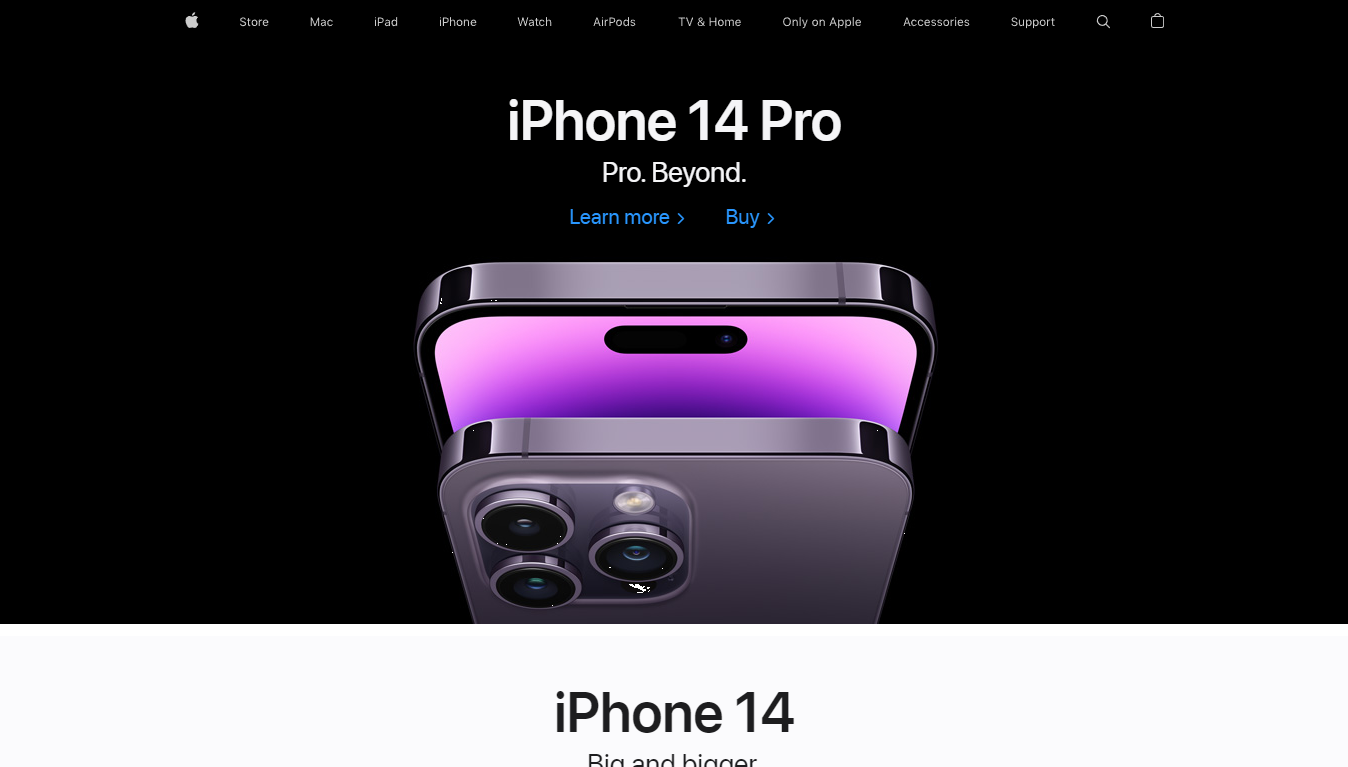On the Apple website, the iPhone 14 Pro page greets visitors with a sleek design against a black background. The headline, "iPhone 14 Pro. Pro. Beyond," emphasizes the advanced capabilities of the device. Below the tagline, there are options to "Learn more" or "Buy" the phone. Featured prominently is a high-resolution image of the iPhone 14 Pro itself. The image showcases the phone's front, where the traditional notch has been replaced with a more elegant, centrally located cut-out for the camera, giving it a cleaner look. The back of the phone also appears in the image, highlighting the triple-camera setup. The text near the image teases with the phrase, "Big and bigger," partially cut off by the edge of the screen.

At the top of the page, a navigation bar with small, readable links allows users to explore other sections such as the Store, Mac, iPad, iPhone, AirPods, Accessories, and Support. There's also a magnifying glass icon for search, and the Apple logo serves as a home button. The picture of the iPhone is positioned at an angle, making it appear as though we are looking down at it from a slightly elevated vantage point. The device looks particularly sleek and shiny, emphasizing its premium design.